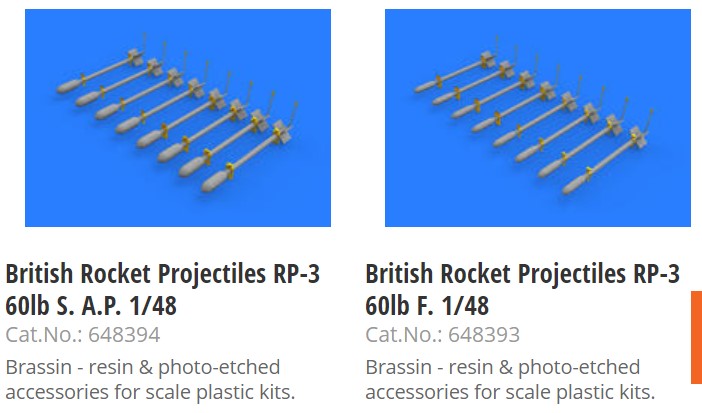The image showcases an advertisement for resin and photo-etched scale plastic model kits featuring British rocket projectiles. There are two side-by-side images with a blue background. Each image displays eight gray projectiles with round tips, arranged diagonally from the upper left to the lower right corner. The left image is labeled "British Rocket Projectiles RP-3 60 lb S.A.P.1/48" and has catalog number 648394, while the right image is labeled "British Rocket Projectiles RP-3 60 lb F.1/48" with catalog number 648393. Both descriptions indicate these are brass, resin, and photo-etched accessories for model kits, likely representing ordinance for scale-model war vehicles or aircraft.